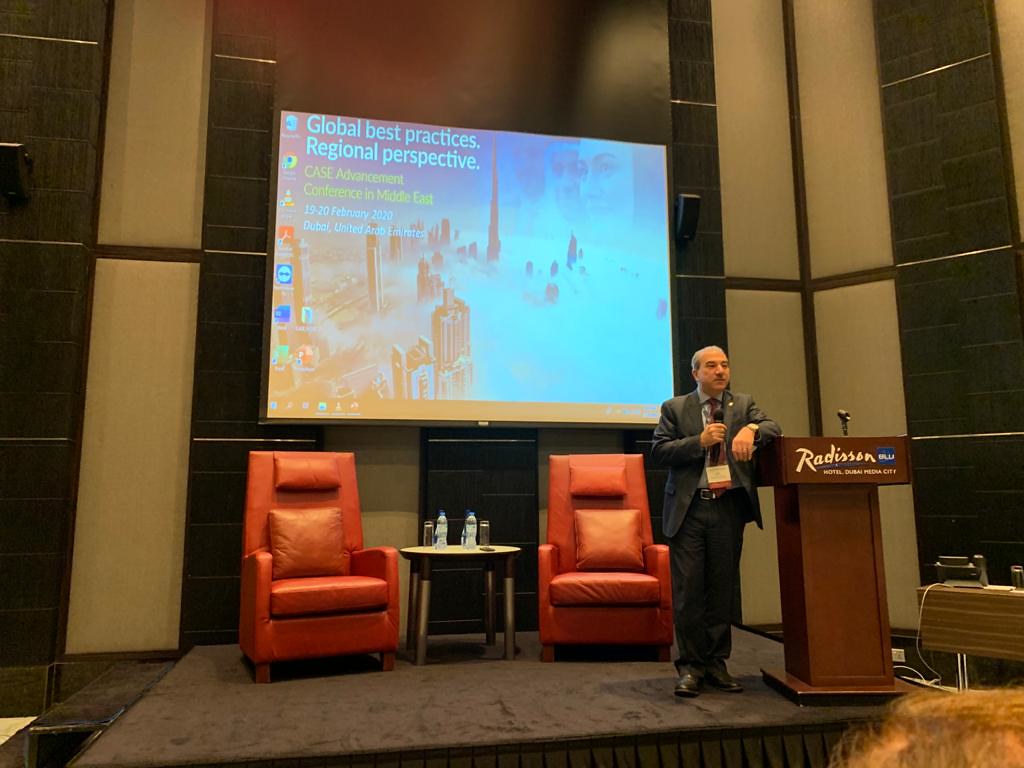The photograph captures a conference setting at a Radisson hotel, focusing on a man in a gray suit, blue shirt, and black tie, wearing a lanyard and holding a microphone. He is leaning against a wooden podium with the "Radisson" logo prominently displayed and a microphone mounted on top. The man is speaking to an audience, positioned centrally on a stage with two orange leather chairs and a round table with water bottles and glasses between them. Behind him, a large monitor displays text reading "Global Best Practices, Regional Perspective," and "Case Advancement Conference in Middle East," framed by a sketch of a cityscape with skyscrapers and clouds. The setting features tall walls and some electrical equipment on a counter to the right. The lower-right corner of the image reveals a hint of another attendee's head, suggesting an audience presence.